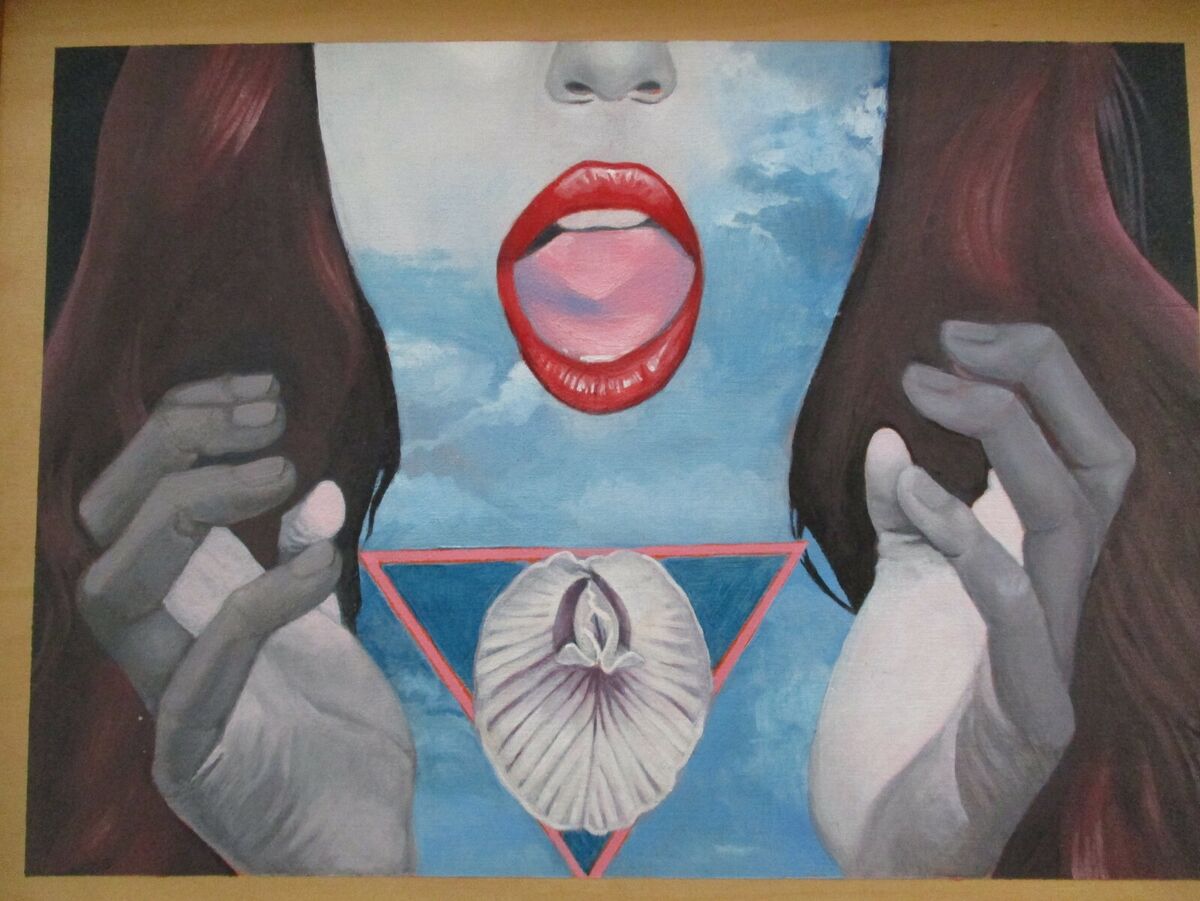The image depicts an abstract and surreal painting of a woman's face. Her skin is an ethereal blend of a blue sky and white clouds, creating a translucent effect. She has long, dark brown hair cascading around her face. Her lips are painted a striking red, and her mouth is open, revealing a pink tongue. Her nose and hands are a grayscale mixture of gray and white. The woman's hands are raised towards her neck, framing an upside-down triangle. This triangle is pink with a blue interior, and within it lies a white form that simultaneously resembles a flower petal, a human heart, and lungs. The intricate design gives the painting a detailed and creative flair, rendered in what appears to be a mix of marker and grayscale graphic design. The abstract elements and the imaginative use of colors and shapes evoke a sense of depth and metaphor within the artwork.